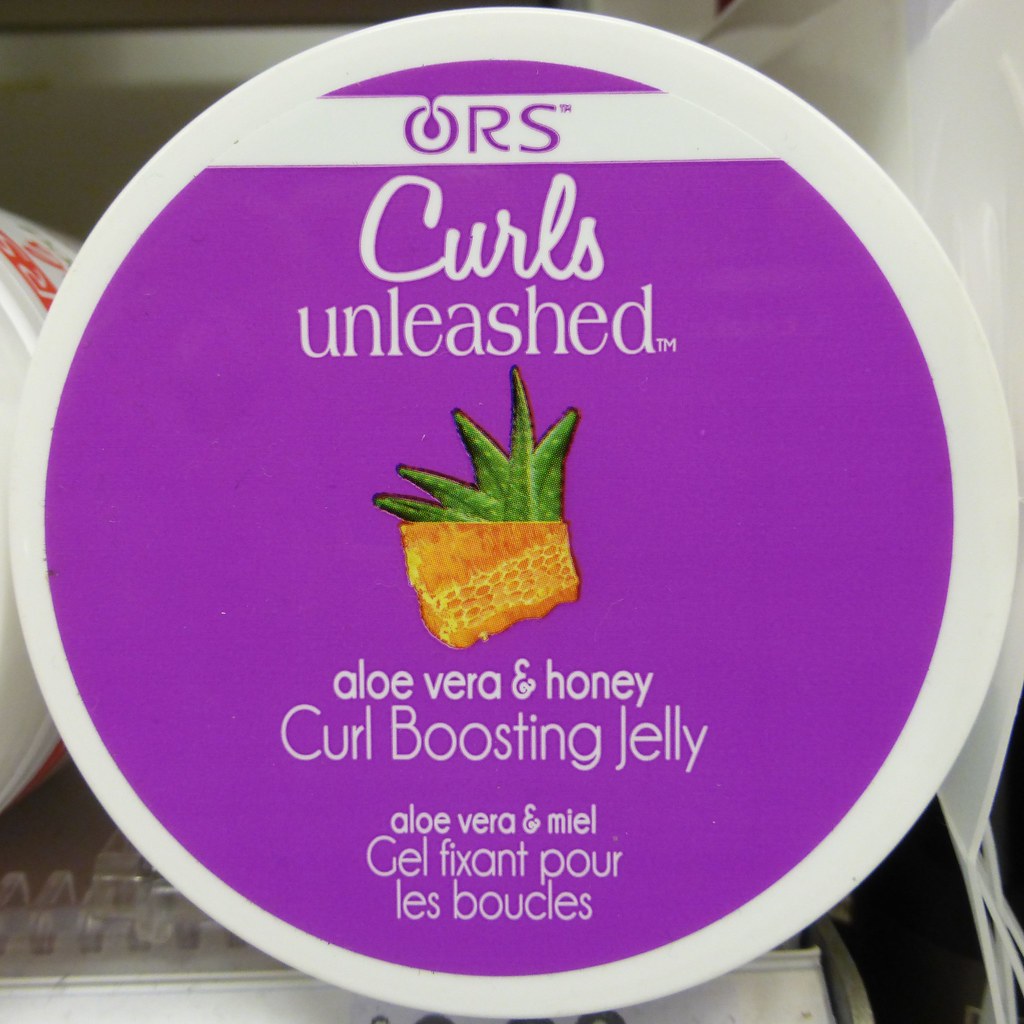The photo features a product prominently displayed on a store shelf. The product is a circular jar with a lid that has a white border and a purple background. On the top of the lid, the brand name "ORS" is displayed in pink lettering, followed by "Curls Unleashed" written with "CURLS" in cursive white font and "unleashed" in regular white font. The central image on the lid depicts an aloe vera plant paired with a honeycomb, symbolizing the main ingredients. Below this image, in white text, are the descriptions "Aloe Vera and Honey, Curl Boosting Jelly" and a French translation, "Aloe Vera et Miel, Gel Fixant Pour Le Boucles." The close-up photograph captures just the upper part of the jar, with its colorful details contrasting against the store shelf where it is placed.